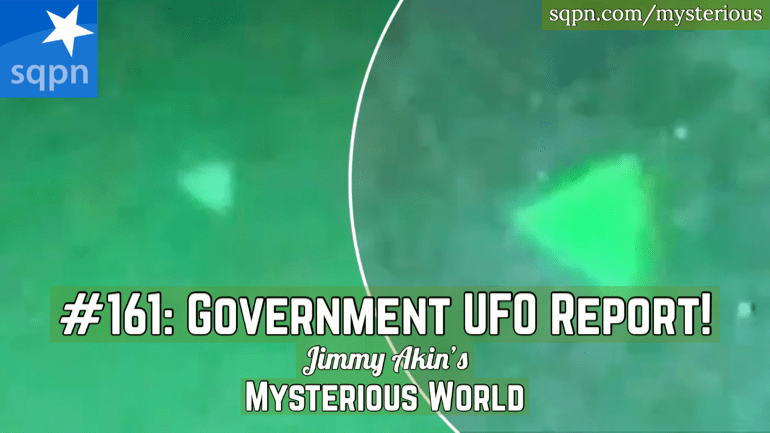The image appears to be a grainy, green-tinted frame, possibly from a video, split into two sections. On the left, a lighter green segment has a blurry, small, bright green triangle, suggesting a view through a night vision lens. The right section zooms in on this triangle, maintaining the green hues but with a darker shade. A thin, semicircular white line separates these two sections. In the top left corner, a small blue logo features a white star with "SQPN" written beneath it in light blue text. The top right corner has a small army green rectangle with the URL "sqpn.com/mysterious" in white text. Centered at the bottom of the image, large white text states "Number 161: Government UFO Report!" Followed by "Jimmy Akin's Mysterious World," each component varying in text size but uniformly white.